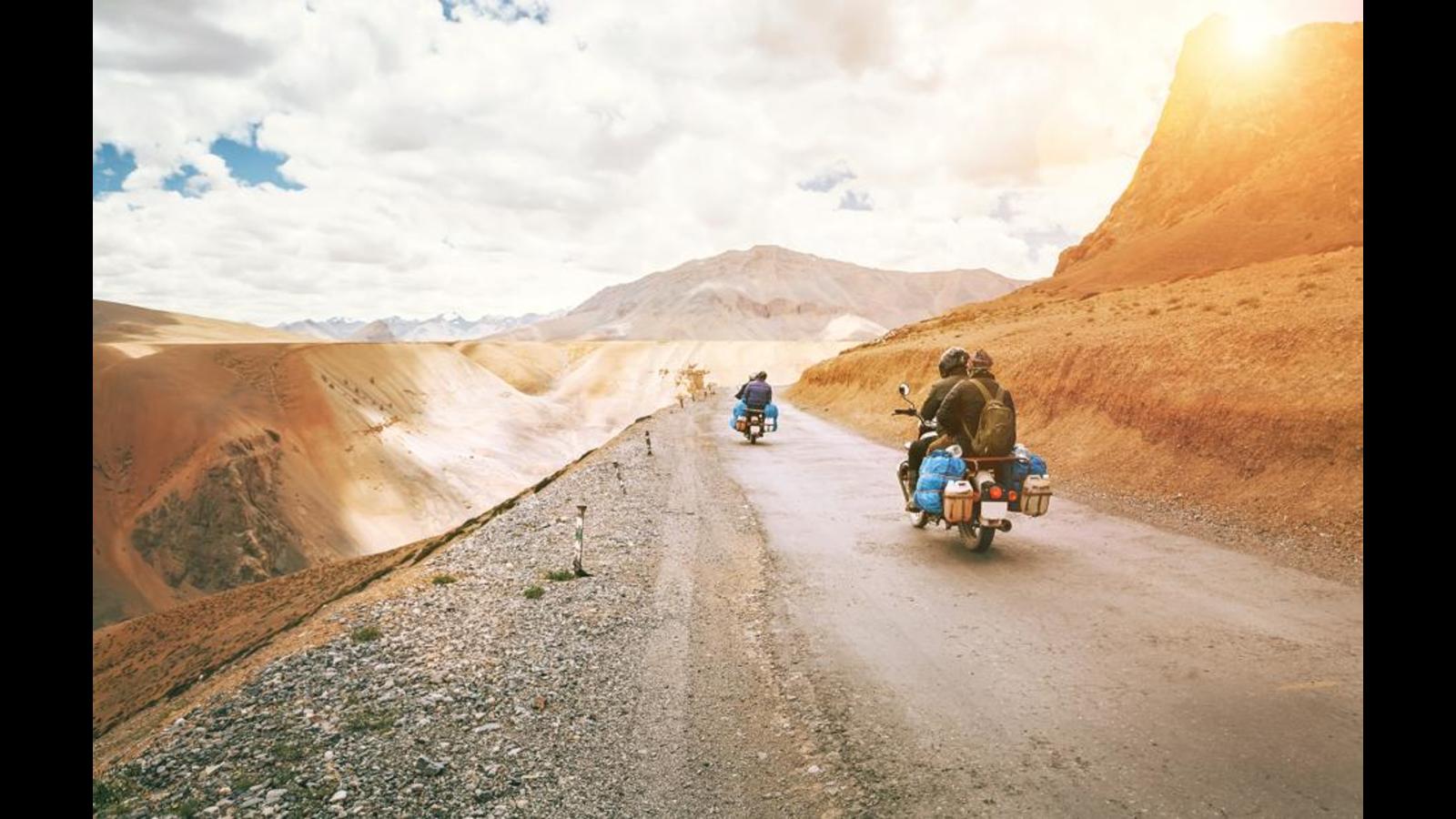In this detailed photograph, two motorcycles with pairs of Euro travelers navigate a narrow, dirt road precariously perched on the edge of a mountain. Laden heavily with packaging, baskets, blankets, and bedrolls, these adventurers ride with an air of determination. The path they're on is bordered by steep mountains: on the right, the jagged peaks ascend dramatically, while on the left, the ground vanishes into a perilous drop, underscoring the treacherous nature of their journey. The landscape is dominated by muted hues—grays, tans, and smoky browns—accentuated by the gritty texture of gravel.

In the backdrop, a vast array of mountains stretches into the horizon, enveloping the scene in a grand, rugged beauty. The sky is a mix of overcast gray with occasional breaks of blue, through which a gentle sunlight filters, emerging from behind the mountain on the top right. This illumination casts a bright, almost harsh light on the scene, contrasting starkly with the surrounding drab colors. Clouds drift heavily overhead, further emphasizing the dramatic and somewhat foreboding atmosphere of their surroundings. This powerful image captures not just the sight of the journey, but its inherent daring and the raw beauty of the untamed landscape.